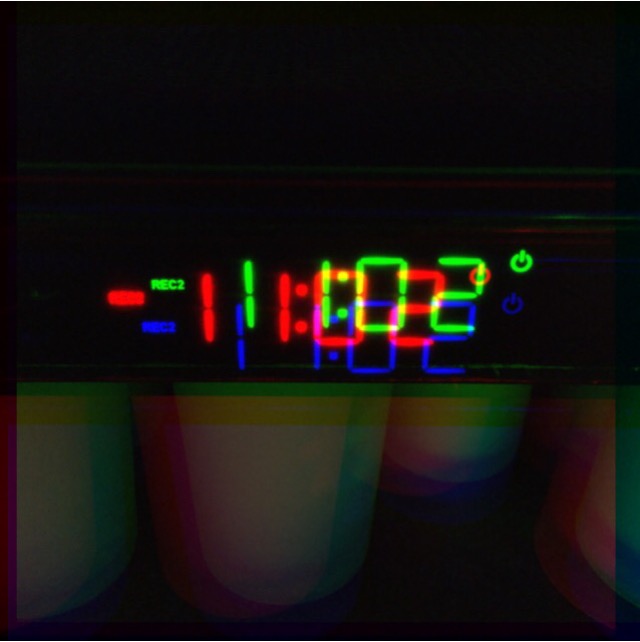This photograph captures a digital clock face displaying a dynamic array of colors, reminiscent of a prism effect. Dominating the right side of the display are three colorful power buttons: a green button, a red button that slightly overlaps with the numerals, and a blue button. These buttons are illuminated digitally, adding to the visual complexity.

On the left side, the clock displays "REC2" in green letters. Adjacent to this, although slightly blurred, the same "REC2" appears in red, and underneath, it repeats in blue.

The time is also depicted in three distinct colors. The red numeral "1" and the blue numeral "1" stand lower than the green numeral "1" at the beginning. A series of colons and numerals follow: a red "1" followed by a colon, a red "0" with a green "1" and blue "1" adjacent, another colon in blue, a green "0", a blue "0", then red, green, and blue "2's" respectively, all contributing to the blended hue effect. The displayed time reads as 11:02, though each color pathway offers a unique way to read and interpret it.

Beneath the numerals, four small white circular objects dot the display, adding subtle detail to the overall composition of this multi-colored digital representation.